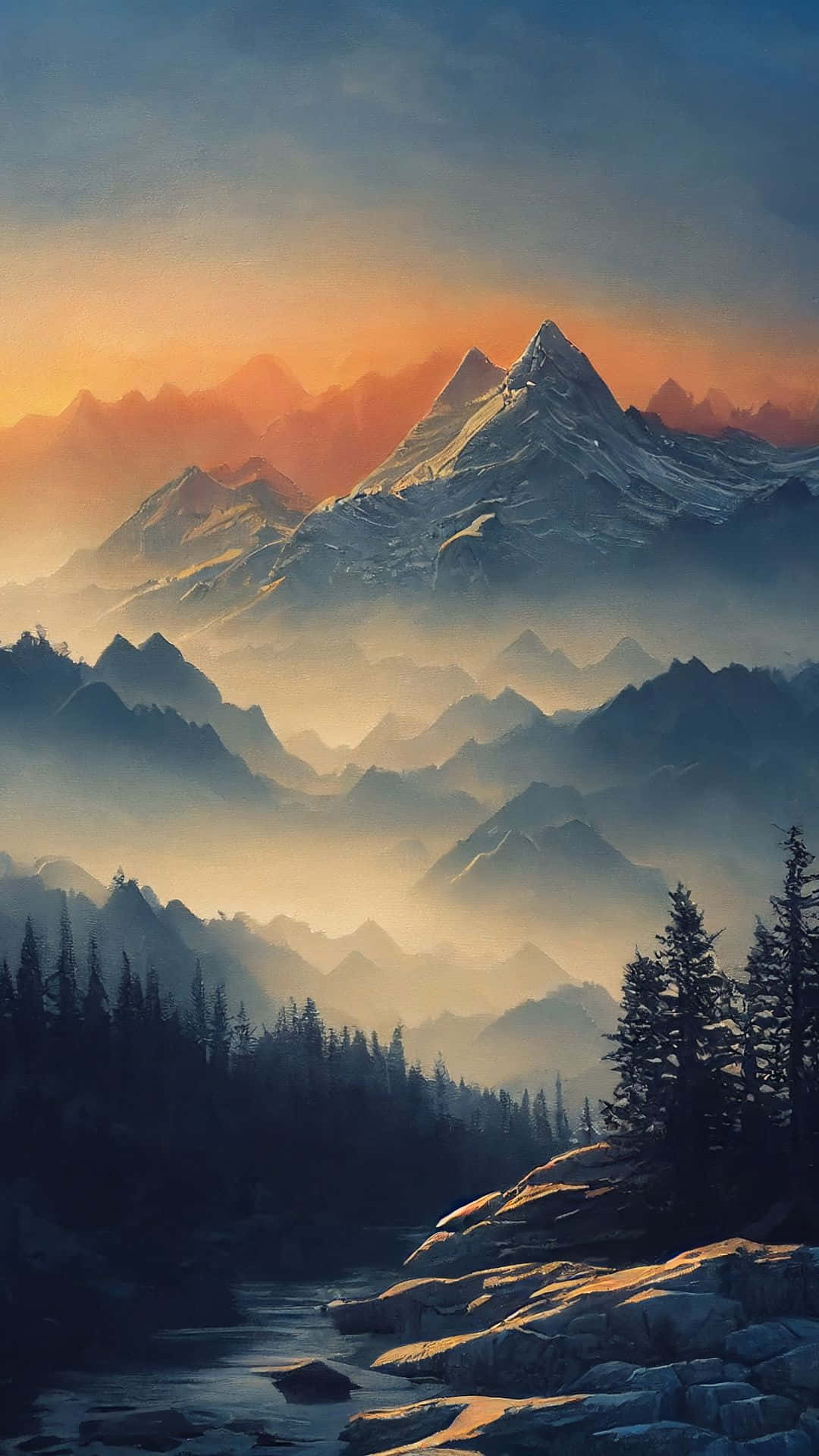In this stunningly picturesque, almost painting-like outdoor scene, the sky at the top is a deep blue, gradually transitioning to a vibrant orange hue, indicating a setting sun. The horizon reveals an extensive mountain range, where the furthest peaks are tinged a peachy orange, fading into gray as they approach. Wisps of clouds or fog hang low, filling the valleys between the mountains. Tall evergreen pine trees flank both sides of the image, with the right side showcasing a shoreline dotted with large boulders. A serene, still stream winds through the landscape, reflecting the tranquil beauty of its surroundings. The overall atmosphere is suffused with a bluish tone, emphasizing the calmness and the natural splendor of the scene.